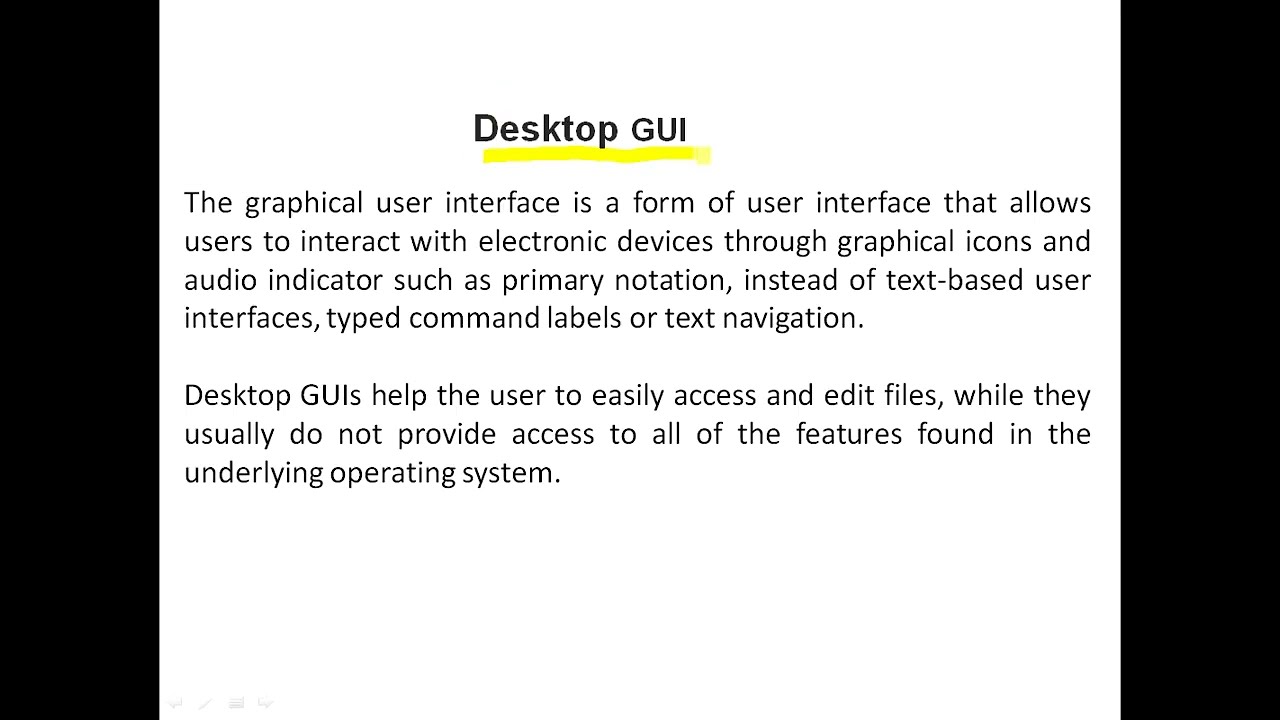The image is a screenshot of what appears to be a PowerPoint presentation slide. The slide features black vertical strips on the left and right sides, framing a white background in the center. At the top of the slide, the title "Desktop GUI" is prominently displayed, with "Desktop" in bold and larger font, and "GUI" in all uppercase letters. This title is underlined with a yellow highlight. Below the title, two paragraphs in black text offer a detailed description of what a GUI (Graphical User Interface) is. The text explains that a graphical user interface allows users to interact with electronic devices through graphical icons and audio indicators rather than text-based interfaces, such as typed command labels or text navigation. It highlights that desktop GUIs help users easily access and edit files but usually do not provide access to all features of the underlying operating system.